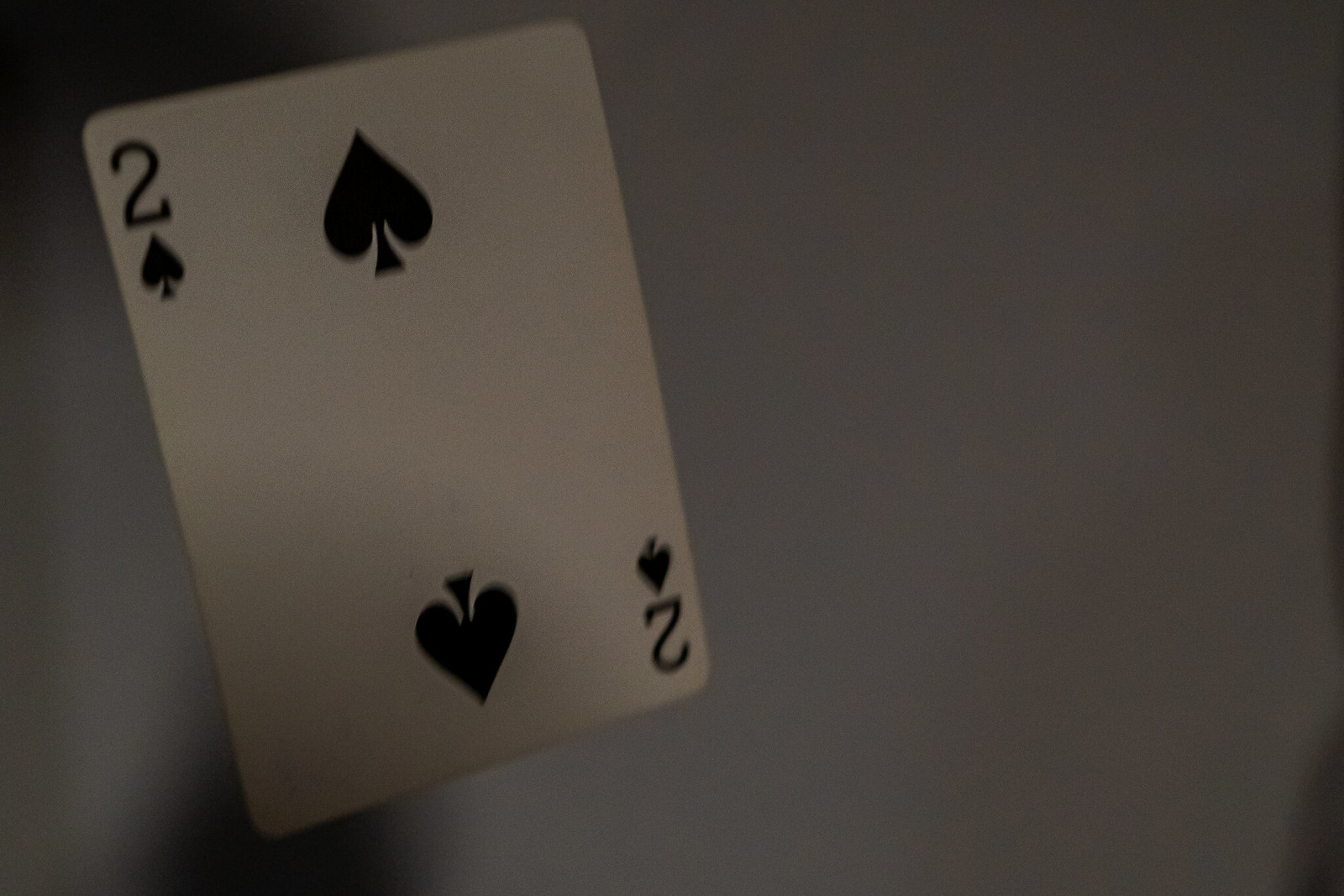In this dimly-lit, low-resolution landscape photograph, a single playing card, the two of spades, takes center stage. Positioned on the left half of the image, the card rests at a precise 45-degree angle to the bottom edge, creating a dynamic yet mysterious focal point. The monochromatic card stands out starkly against a murky grey background, which is muddled with indistinct shadows of unknown origin. The bottom left third of the playing card is shrouded in a subtle shadow, caused by a diffuse light source that casts soft, indistinct patterns. The right side of the image remains vacant, revealing only a darker portion of the grey background and a hint of shadow in the bottom right corner, whose source is equally unclear. The most prominent shadow exists on the bottom left corner of the playing card, heightening the overall sense of ambiguity and obscurity in the scene.